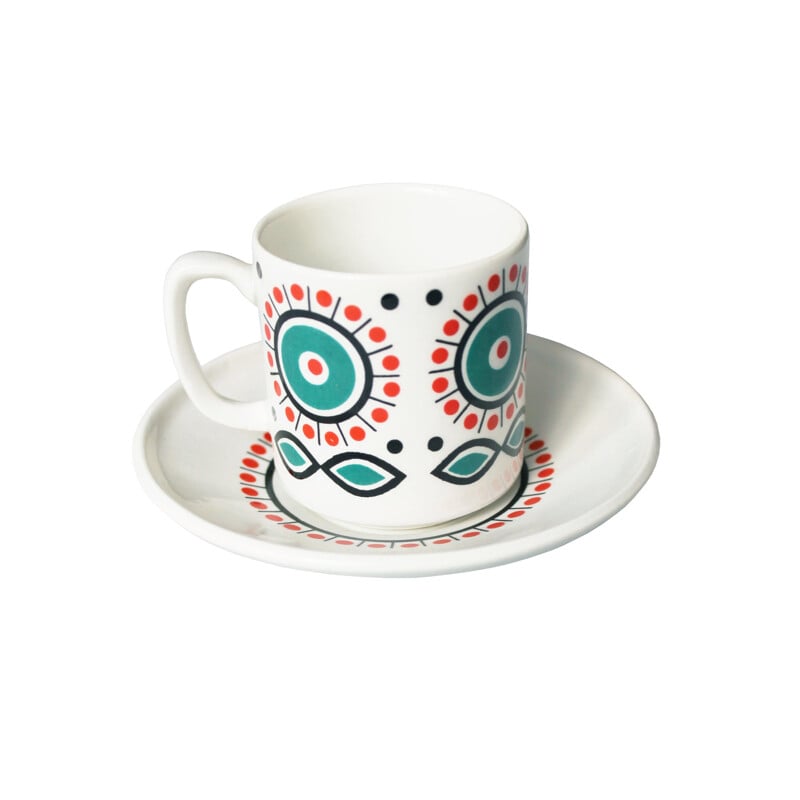A detailed photograph features a white mug alongside a matching saucer, set against a clean white background. The saucer, positioned centrally, showcases an intricate design: a dark circle at its core, radiating perpendicular lines interspersed with red dots. The white mug mirrors this pattern, with added nuances; inside the mug, a pink circle encircles a red dot, and beneath it, there's an eye-like design. Though empty, the mug stands out with its smooth surface and generously sized handle, inviting touch and use.